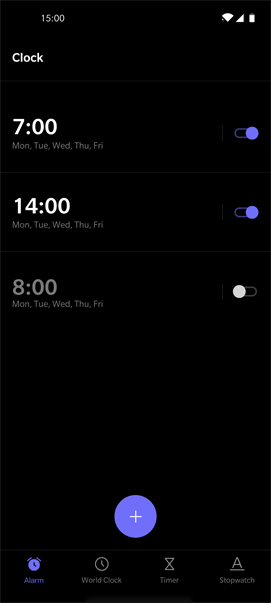This color image appears to be a screenshot taken from a smartphone, displaying the device's 'Alarms' page. In the top left corner, there is a time stamp showing "15:00" in white text. The battery indicator, also located at the top of the screen, suggests that the phone is fully charged.

The background of the screenshot is solid black, and all text is displayed in white for contrast. The page lists three alarms. The first alarm is set for 7:00 AM from Monday through Friday and is currently turned on. The second alarm is set for 14:00 (2:00 PM), also from Monday through Friday, and it too is turned on. The third alarm is for 8:00 AM, similarly set for the weekdays, but this one is currently turned off.

At the bottom of the screen, there's a purple button with a plus ("+") symbol in the center, indicating the option to add more alarms. In the lower navigation menu, four icons are visible: the alarm function on the far left, followed by the world clock, timer, and stopwatch functions.